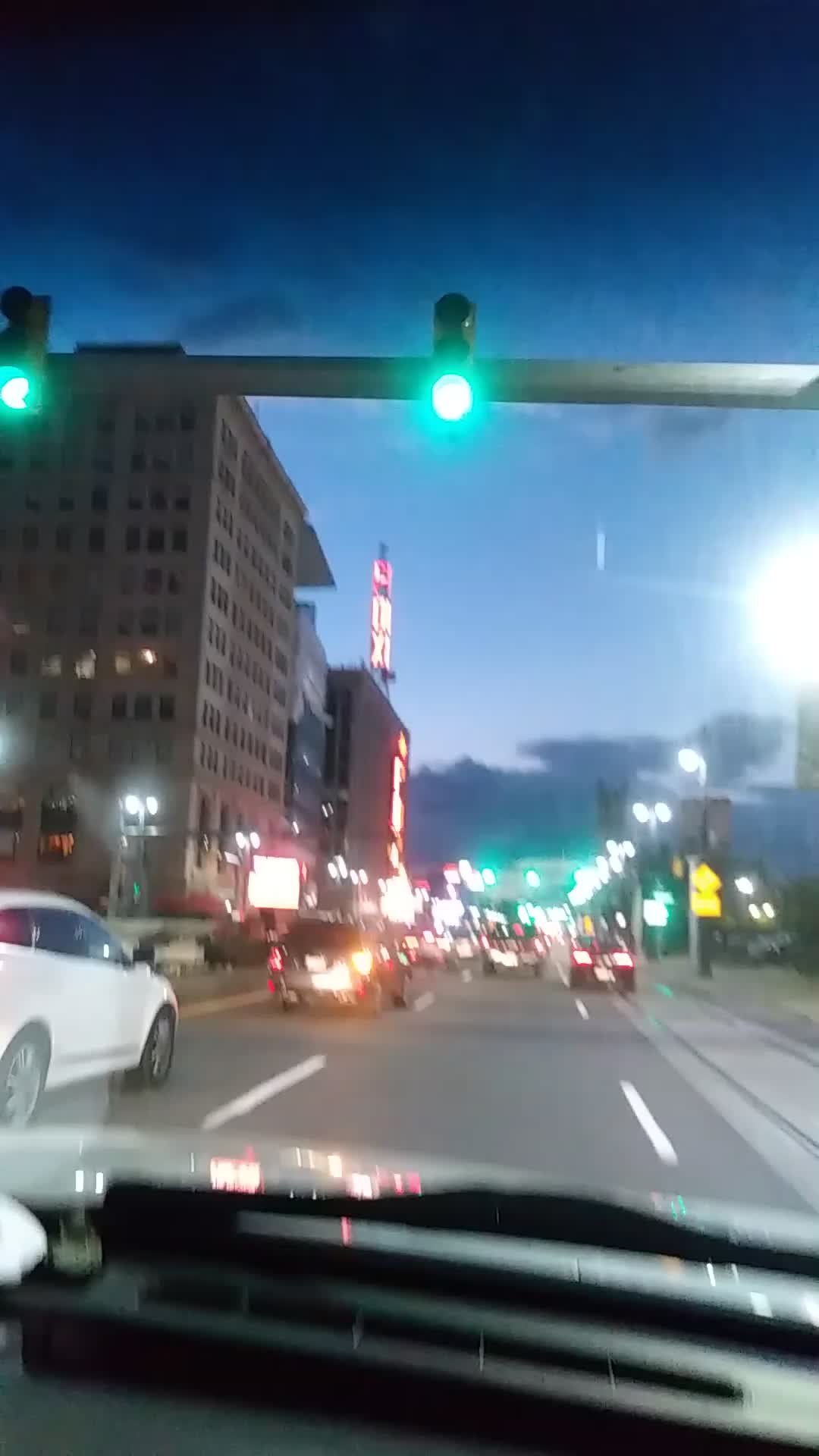This photo captures a dynamic scene of city driving at twilight. The sky is a blend of deep blue and pink hues, suggesting either sunset or sunrise, with dark clouds beginning to envelop the colorful backdrop. A green traffic light hangs directly above the scene, indicating the way forward. Multiple vehicles populate the road with five cars ahead, including a white car fairly close on the left, a black SUV merging into the lane, a truck further ahead, and a black car to the right. The cityscape features a large building with most of its lights off, hinting at the end or start of the day. The streets are illuminated by several green traffic lights and numerous street lamps lining the right side of the road. Neon signs from buildings on the left add to the urban atmosphere. The image is blurry, heightening the sense of motion through the bustling city at this transitional time of day.